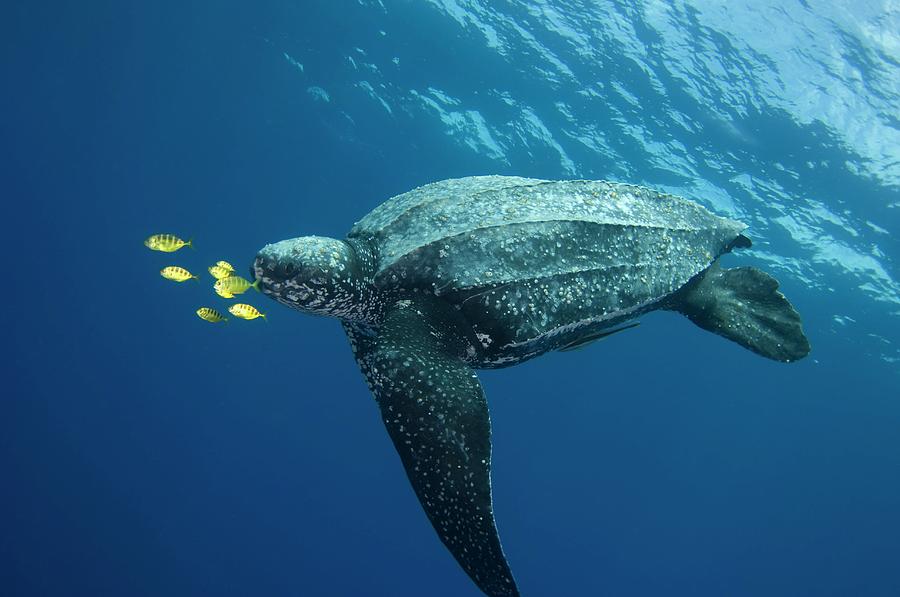In this detailed underwater scene, a majestic, weathered sea turtle with a shell resembling rusted stone glides through the deep blue ocean. The turtle, covered in white spots and ridged sections on its shell, suggests its age and past encounters with barnacles. Prominent fins extend below it, with a noticeably large green fin with white spots along the left side. Underneath its head, more white spotting is visible on its chin and neck. In the upper right, sunlight penetrates the water, creating a light blue shimmer and highlighting the vast, empty abyss to the left. Swimming just inches in front of the turtle's head, a school of about six to seven small yellow fish, some with black stripes, moves in unison with the turtle, adding vibrancy to the serene blue expanse.